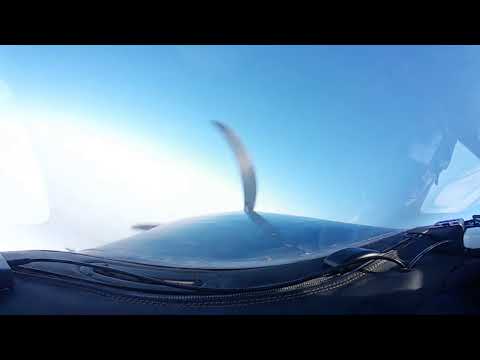This image captures a close-up view taken from the cockpit of a single-engine airplane in mid-flight, emphasizing the silver propeller set against a backdrop of a blue sky with white clouds scattered below. The black cockpit dashboard stretches across the bottom of the image, complementing the blurred motion of the propeller which gives a sense of the plane's active flight. The plane appears to have a black hood, and there's a noticeable glare from the sun in the sky, casting a white light to the left. Reflecting various interpretations, there seems to be a black, curving element that some might identify as a zipper on a bag, adding a bit of confusion and potential clutter within the cockpit area. Additionally, subtle details such as a possible heart shape formed by an airplane's path in the sky and some items like wires or paper suggest a less pristine, more lived-in interior, potentially hinting at a real-life candid shot rather than a professional or highly stylized photograph.